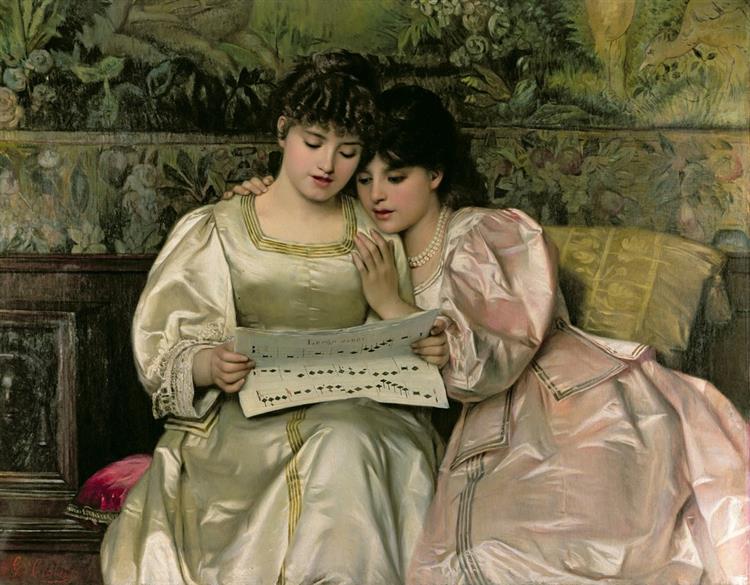This detailed painting captures a serene moment between two young women, likely sisters or close friends, who are seated closely on a cozy love seat in an elegantly decorated living room. The one on the left, dressed in a satin gown with hues of light lime and white, has beautifully curled hair, a girlish face, and red lips. She holds a piece of paper that appears to feature musical scales or geometric progressions. The woman on the right, adorned in a shimmering dress with a pinkish-orange tint, leans on her companion's shoulder, gazing intently at the paper. Her darker hair and poised demeanor complement the scene. The background reveals a rich, brown wainscoted wooden wall rising halfway up, topped with a flowery green tapestry featuring intricate designs of plants, birds, and trees. A carved walnut dresser with a face motif adds to the room's refined ambiance. Completing the setting, a golden pillow rests behind the right-hand woman, accentuating the painting's overall warmth and intimate atmosphere.